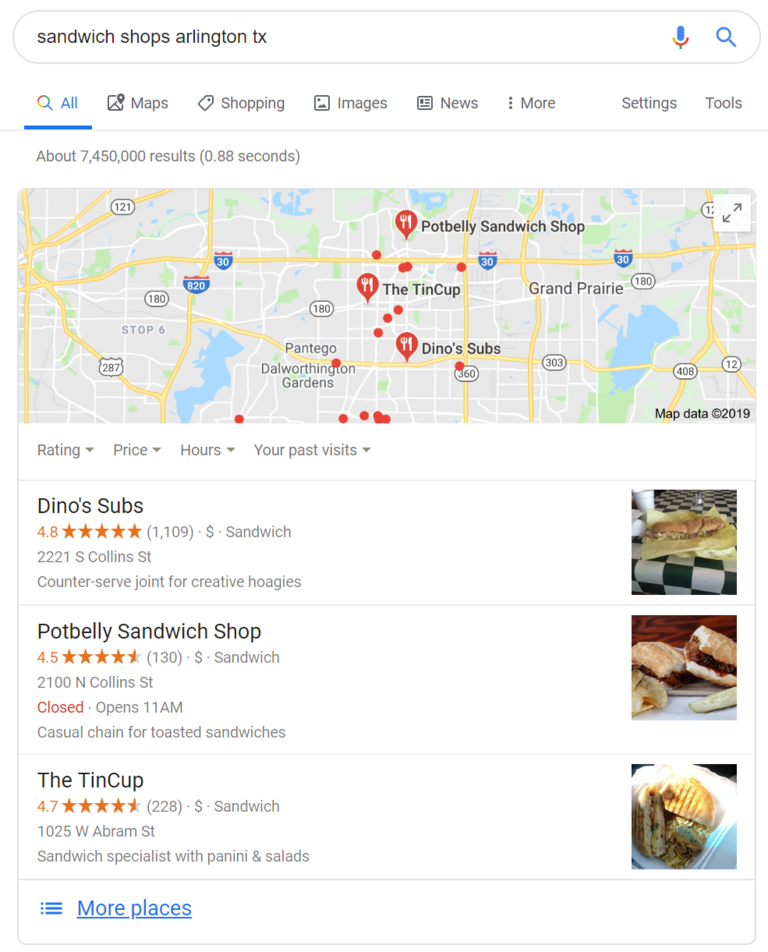**Detailed Caption:**

The image portrays a Google search results page specifically for "sandwich shops in Arlington, TX." The top portion showcases the Google search bar, filled with the query "sandwich shops Arlington TX," accompanied by a blue microphone icon and a blue magnifying glass icon to its right. Below the search bar, there are several navigational options: the "All" tab highlighted in blue, and adjacent to it, other options in gray which include "Maps," "Shopping," "Images," "News," "More," and an array of settings and tools on the far right.

Underneath these options, a thin gray bar displays the search results summary: approximately 7,450,000 results in (0.88 seconds). Dominating the central part of the image is a large rectangular map of Arlington, Texas, marked with multiple red dots representing sandwich or sub shops. The map's background features standard map details including yellow highlighted highways and expressways, labeled state highways, US highways, parks in green, and blue lakes. Each red dot aligns with search results listed below the map. The lower right corner of the map contains a “Map Data Copyright 2019” notice.

Beneath the map, there are sorting options that include "Rating," "Price," "Hours," and "Your Past Visits," each accompanied by a gray down-facing triangle for additional selections.

Following these options are detailed listings of three sandwich shops:

1. **Dino's Subs**
   - Rating: 4.8 out of 5 (fully highlighted in orange)
   - Reviews: 1,109
   - Price: $
   - Category: Sandwich
   - Address: 2221 S Collins Street
   - Description: A counter service joint known for creative hoagies.
   - Thumbnail: A small image of a hoagie on a checkered tabletop with a white cup.

2. **Potbelly Sandwich Shop**
   - Rating: 4.5 out of 5 (four and a half stars shaded in orange)
   - Reviews: 130
   - Price: $
   - Category: Sandwich
   - Address: 2100 North Collins Street
   - Status: Currently closed (opens at 11 AM)
   - Description: A casual chain offering toasted sandwiches.
   - Thumbnail: A small image of sandwiches with meat on a table with a red background.

3. **The Tin Cup**
   - Rating: 4.7 out of 5 (four and a half stars highlighted in orange)
   - Reviews: 228
   - Price: $
   - Category: Sandwich
   - Address: 1025 W Abrams Street
   - Description: Specializes in panini and salads.
   - Thumbnail: A small image displaying a panini sandwich against a white napkin backdrop.

Below these listings, there is a blue icon with three black blue dots and three horizontal bars, next to the underlined hyperlink "More places."